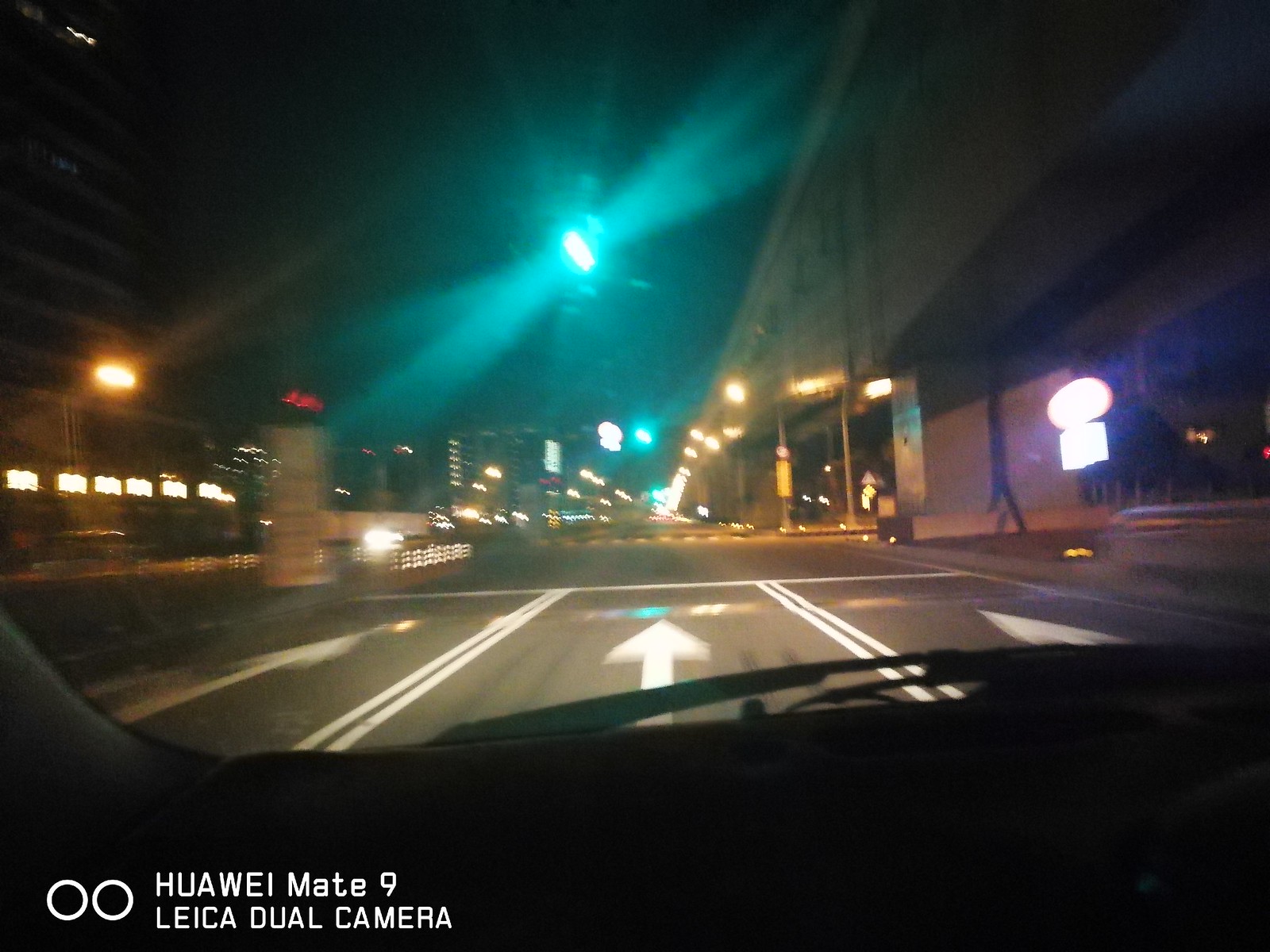The image is a blurry, nighttime dashboard cam photo, likely taken from the driver’s side of a vehicle, possibly attached to the sun visor. The photo depicts a wide, three-lane city street, delineated with white lane markers and forward-pointing arrows on each lane. There is an illuminated green traffic light at the center top of the image. The road is lit by numerous streetlights and features reflected lights and signs, possibly due to the camera flash. On the right side of the road, there's a large bridge-like structure, possibly part of a public transit system, supported by concrete columns and emitting lights. In the far background, a skyscraper is visible, indicating a densely populated area. To the left of the image, there’s a corporate or brick building with white trim. The bottom-left corner of the image shows the logo “Huawei Mate 9 Leica dual camera” alongside two circular outlines. You can also see a windshield wiper and a portion of the car’s dash, emphasizing the in-motion capture of this urban night scene.